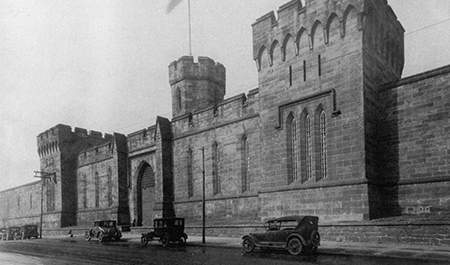This image depicts a photorealistic black and white photograph with a focus on a large stone-brick wall extending from right to left at an angle, drawing the viewer's eye from the foreground into the background. The right side of the wall, being closer to the viewer, prominently showcases intricate details including many elongated windows and a central gate that is slightly offset to the left of center. Flanking the central gate are two imposing guard towers, while further behind them looms a larger, roundish stone tower adorned with a parapet and a flagpole, from which a banner hangs. Parallel to this impressive medieval structure runs a dark-colored street lined by several early 1900s T-model cars, some open and some with covers, all uniformly dark in color. The scene is set under a somber dark gray sky, enhancing the historic and somewhat nostalgic atmosphere of the photograph. The dimensions of the photo are approximately three to four inches wide by two inches high, contributing to its old-fashioned charm.